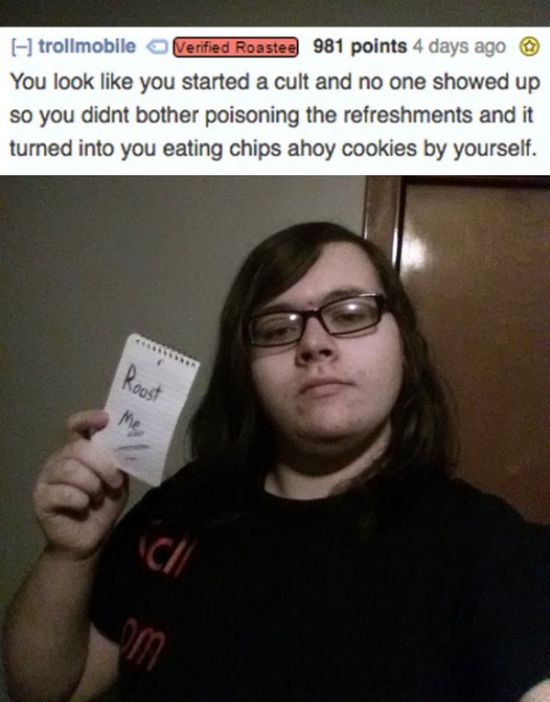A social media post by user Tromobile, labeled as a verified roaster with 981 points from four days ago, features the humorous caption: "You look like you started a cult and no one showed up so you didn't bother poisoning the refreshments and it turned into you eating Chips Ahoy cookies by yourself." Below this, an image depicts a young person with shoulder-length brown hair and rectangular eyeglasses, wearing a black t-shirt with red or orange writing on the right side. The person holds up a small notepad in their right hand with a handwritten sign that humorously misspells "Roast Me" as "Roost Me." They have a neutral expression and are posed in front of a solid brown door and a gray or possibly white wall in a dimly lit room.